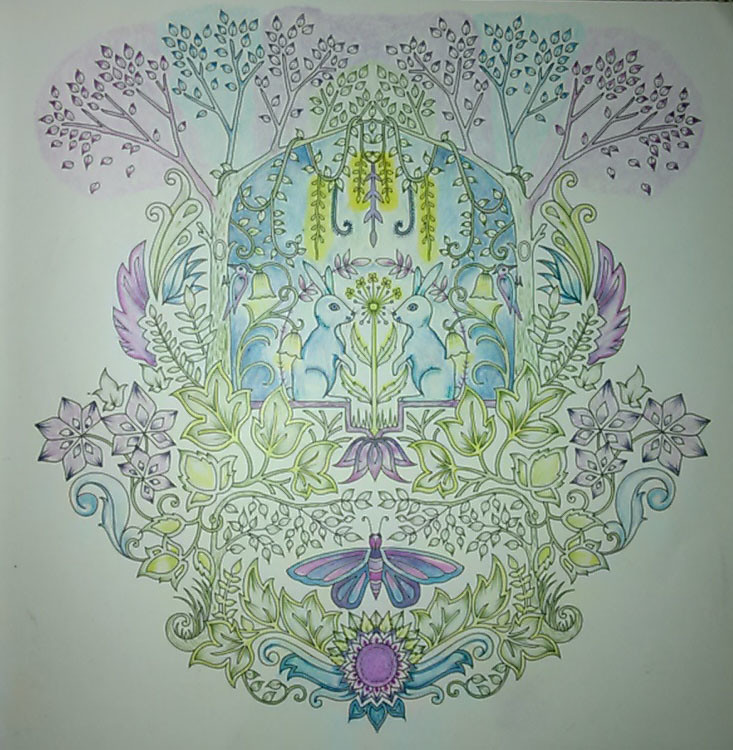The image is a vibrant and detailed drawing set against a cream background, incorporating an array of pastel colors such as pink, turquoise, yellow, light blue, green, and purple. At the center, two blue rabbits face each other, separated by a tall flower. The entire scene is richly embellished with flora and fauna.

Surrounding the rabbits is a beautiful arch formed by two trees adorned with intricate, droplet-shaped leaves in shades of pink, light green, light blue, yellow, and purple. Hanging from the arch are delicate yellow flowers resembling a chandelier.

Beneath the rabbits, a purple butterfly with blue shading is depicted amidst swirling green ivy and purple flowers, contributing to a lush, organic design. Below this, the ivy intertwines with a purple jewel-like flower that rests above a decorative purple trim. The bottom section of the drawing features more foliage, with light cream petals and teal ribbons framing a central purple flower seed adorned with pointy, light green petals.

Overall, this artwork boasts an intricate balance of delicate plant details and vivid, colorful highlights, creating a captivating and harmonious scene.